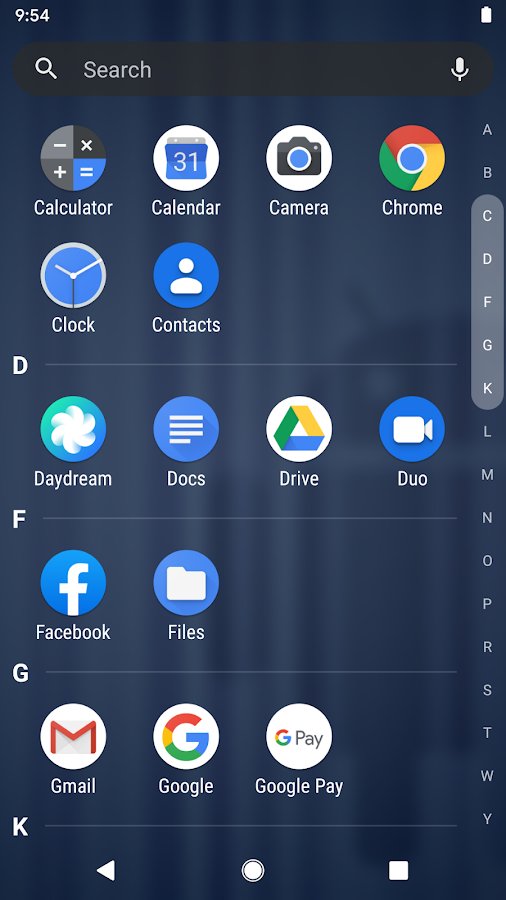This detailed screenshot captures the home screen of a mobile device. The status bar at the top displays the time at 9:54 and a battery status at 4%. The background features a dark blue, blurry abstract image. At the bottom, there are three navigational buttons: a backwards triangle (back button), a circle (home button), and a square (recent apps button). Prominently displayed at the top of the home screen is an empty search bar equipped with a microphone icon, enabling voice search functionality. The person in the image is navigating through the phone's applications, which are alphabetically organized along the right-hand side with a scrolling bar. The visible sections on the screen are marked by their respective letters: C, D, F, and G, indicating the grouped apps within each alphabetic category.